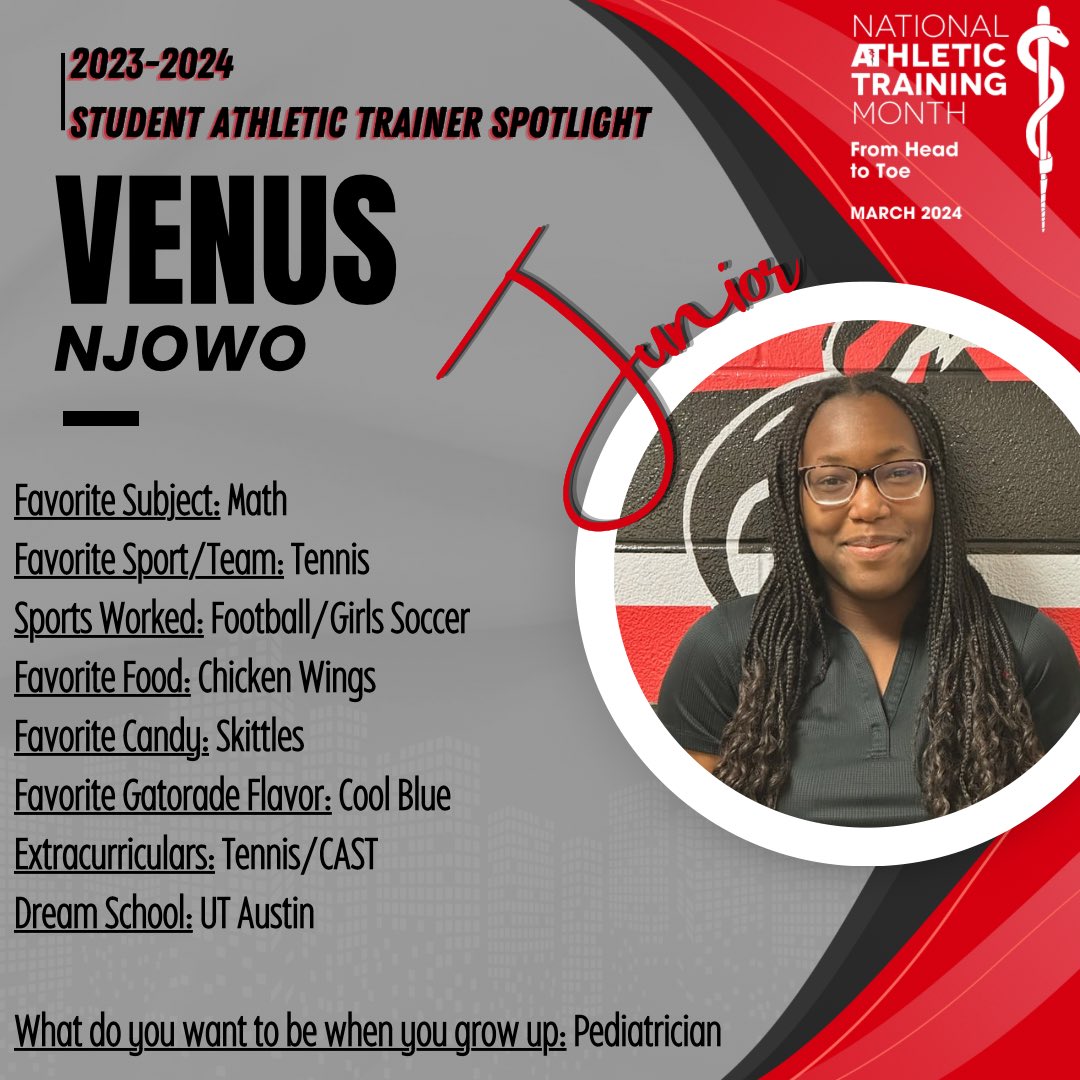The poster for the 2023-2024 Student Athletic Trainer Spotlight features a detailed profile of Venus Njowo, an African-American junior with braided hair and glasses, smiling in a semi-professional black polo shirt. The poster is part of National Athletic Training Month, marked from head-to-toe in March 2024. Venus stands against a painted concrete block wall, possibly adorned with her school's athletic logo in red, white, and black colors. Her profile includes a variety of personal favorites and activities: favorite subject is math, favorite sport is tennis, sports worked are football and girls' soccer, favorite food is chicken wings, favorite candy is Skittles, and favorite Gatorade flavor is Cool Blue. She participates in tennis and the cast club and dreams of attending UT Austin. At the bottom, it reveals her aspiration to become a pediatrician. The poster also includes an icon of a snake wrapped around a pole, symbolizing medical training.